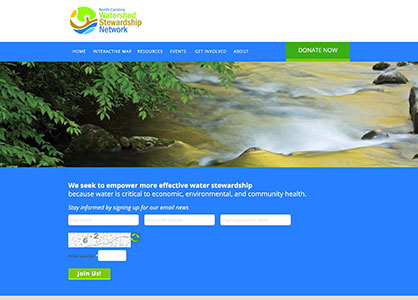The image displays a vibrant web page design characterized by bright blue and white hues. Prominently featured in the upper half of the page is a photograph showcasing the leaves of a tree next to the rushing rapids of water. The water in the image exhibits a blend of light yellow, gray, and white tones, with dark gray rocks visible to the right. At the top of the web page, the logo stands out—a circular emblem featuring green, brown, light blue, and dark blue colors. Adjacent to the logo, "Watershed" is written in green, "Towards Ship" in brown, and "Let's Walk" in blue.